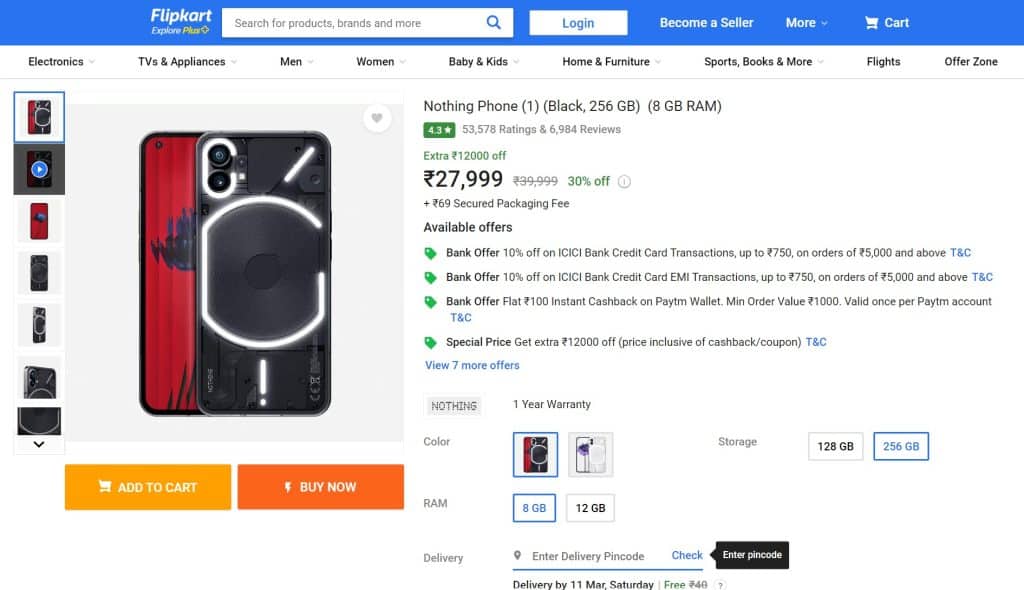The image depicts a section of the Flipkart website interface showcasing a featured product. At the top, a large blue banner displays the text "Explore Plus." To the right of this banner is a white section containing a search bar with the placeholder text "Search for products, brands, and more." Adjacent to the search bar are options to "Login," "Become a Seller," "More," and the "Cart" icon.

Below this header, several navigation tabs are visible, including "Electronics," "TVs & Appliances," "Men," "Women," "Baby & Kids," "Home & Furniture," "Sports," "Books & More," "Flights," and "Offer Zone."

The main section features a prominent image of a smartphone. The phone's rear is black with white lights, while the front is red. To the right of the image is a description of the phone: "Nothing Phone 1, Black, 256 GB, 8 GB RAM." This is accompanied by a green rating indicating "4.3 stars," based on "53,578 ratings and 6,984 reviews." The price is displayed as "₹27,999," with a notable "30% off" discount. Below the price, the text "Available Offers" is followed by a list of four offers, including bank-related promotions.

At the bottom of this section, options to customize the phone's color, RAM, storage, and delivery preferences are available. Two buttons are displayed for purchasing actions: a yellow "Add to Cart" button on the left and an orange "Buy Now" button on the right.